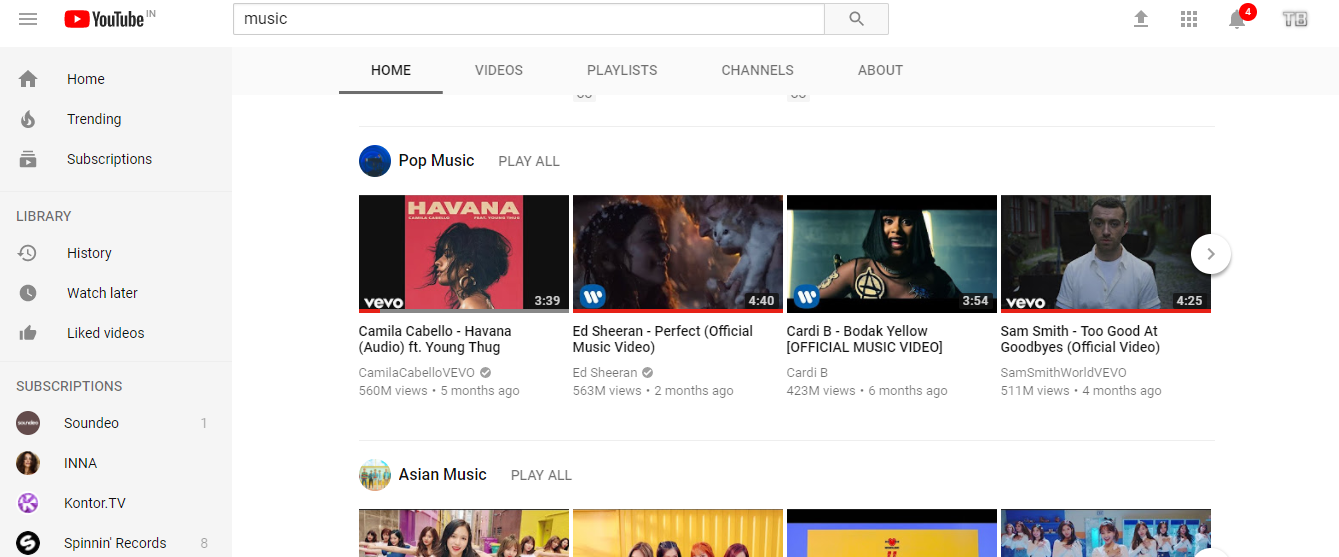This is a detailed description of a screenshot taken from the YouTube homepage in light mode on a desktop or laptop computer. In the upper left corner, the YouTube logo is visible, with the India regional indicator. Adjacent to the logo is a hamburger menu for additional settings. The center top of the screen features a search bar with the word "music" entered and a search button next to it. Following the search area are an upload button, a sort button, a notifications button, and a user channel icon button.

Below this primary toolbar, there is a vertical navigation column starting with buttons for "Home," "Videos," "Playlists," "Channels," and "About." Further down, a "Pop Music" playlist category is highlighted with a "Play All" option, showcasing popular tracks like Camila Cabello's "Havana," Ed Sheeran's "Perfect," Cardi B's "Bodak Yellow," and Sam Smith's "Too Good at Goodbyes." Nearby, there is also an "Asian Music" category, although it is partially cropped off the right side of the screen.

On the far left-hand side, another vertical column provides quick access to various sections, including "Home," "Trending," "Subscriptions," and "Library." The Library section includes links for "History," "Watch Later," and "Liked Videos." The screenshot also reveals a list of subscriptions, featuring channels such as Soundio, Inna, Contour.TV, and Spinning Records. The entire screenshot is displayed in a widescreen landscape format, characterized by a white background with black text due to the light mode setting.